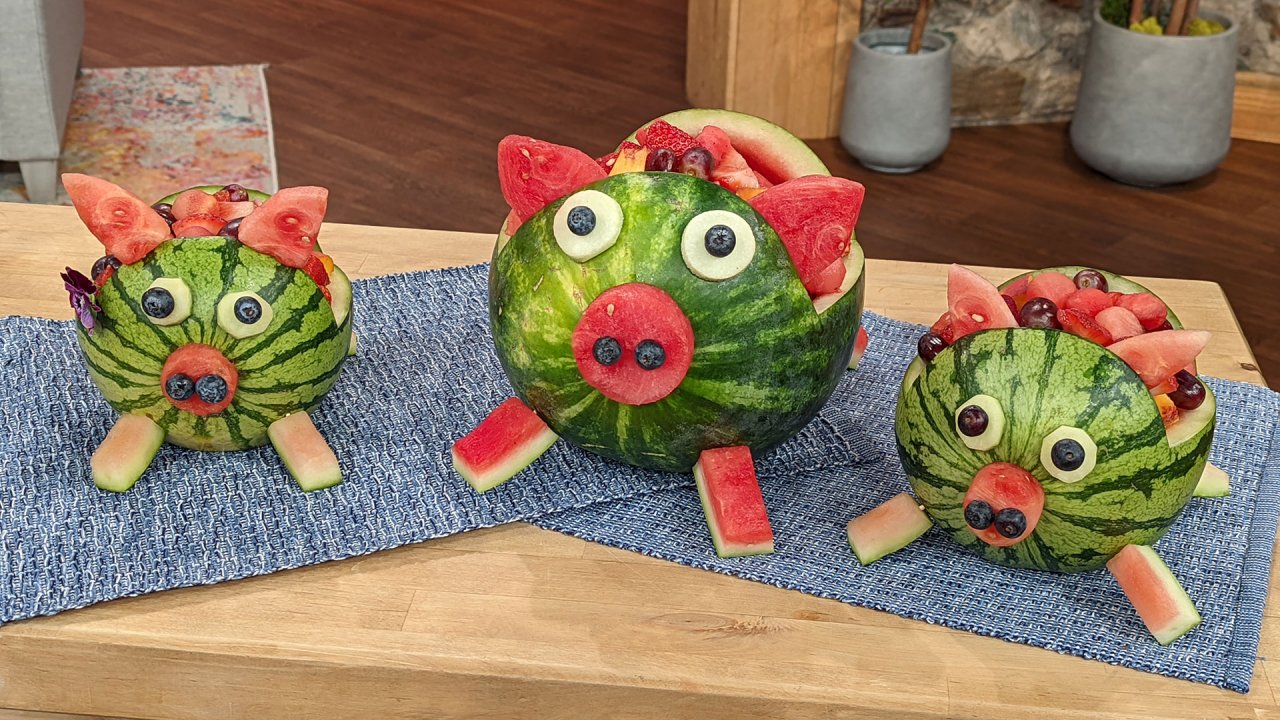In this photo, we see an artistic display featuring three watermelon carvings that have been creatively arranged to resemble cartoon pigs. Each pig is intricately crafted using parts of the watermelon: the ears, nose, and legs are fashioned from watermelon slices, while the eyes and nose incorporate blueberries and possibly slices of bananas. The watermelon pigs function as fruit bowls, with their backs open to reveal an assortment of fruits inside. They are positioned in a row on a table covered with a blue denim-like fabric or gray placemats atop a pale wood-colored surface. The setting is a modern interior, evidenced by the background which includes potted plants, a dark wood floor, a rug, part of an upholstered chair, and the overall ambiance of a stylish living space. The colors in the image range from various shades of green, red, and blue to white, tan, and darker browns, showcasing a vibrant and detailed scene.